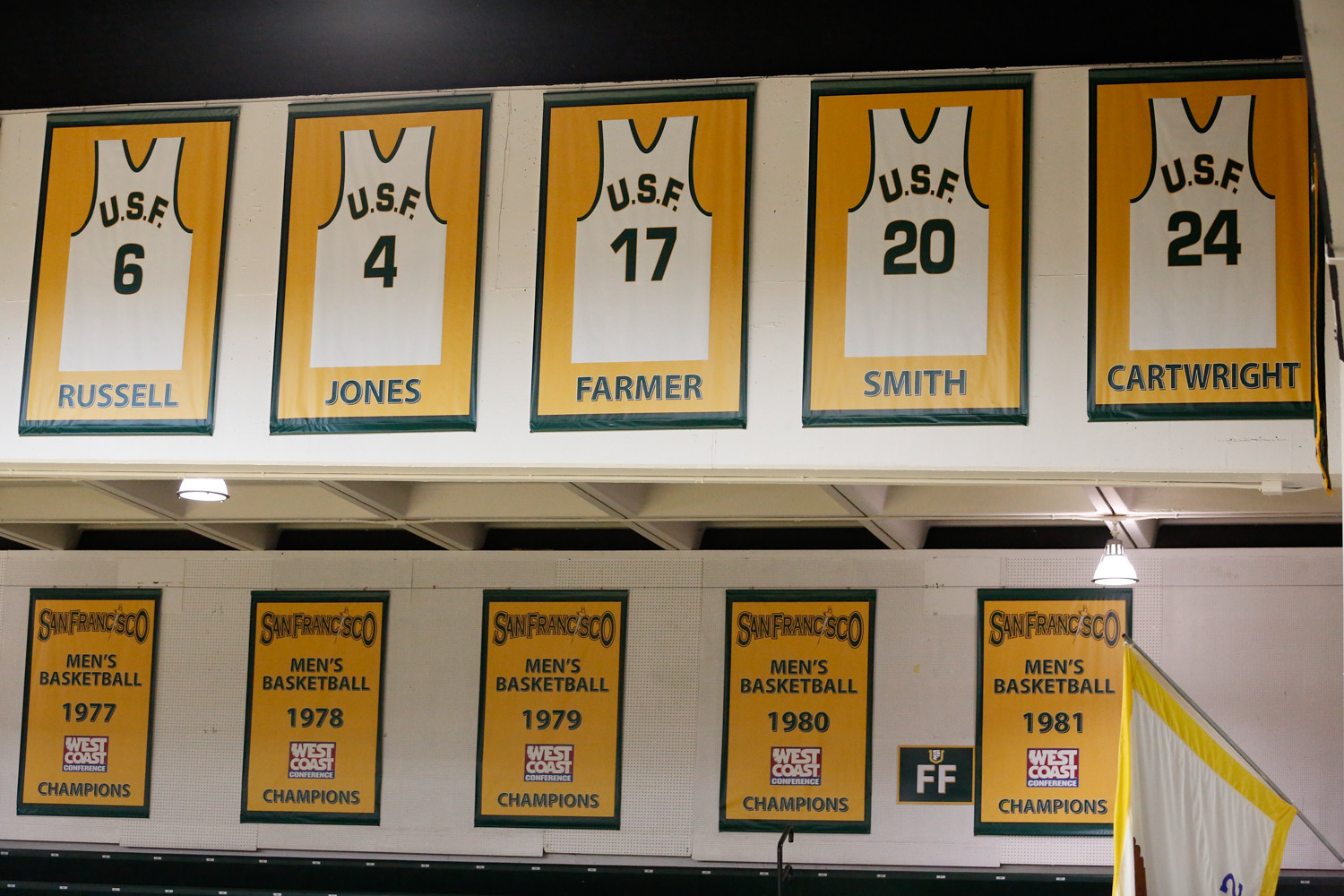The image depicts a display of framed sports jerseys on a white wall in what appears to be a sports gymnasium. The jerseys are white with green trim on the neck and sleeves, displayed on a yellow background and encased in green frames. From left to right, the jerseys read: USF 6 - Russell, USF 4 - Jones, USF 17 - Farmer, USF 20 - Smith, and USF 24 - Cartwright. Below the jerseys, there are framed posters with yellow backgrounds announcing the achievements of the San Francisco Men's Basketball team, listing the years 1977 to 1981 as West Coast champions. In the bottom right corner, partially cut off, there is a flag with a yellow border, white center, and a brown wing extending outward.